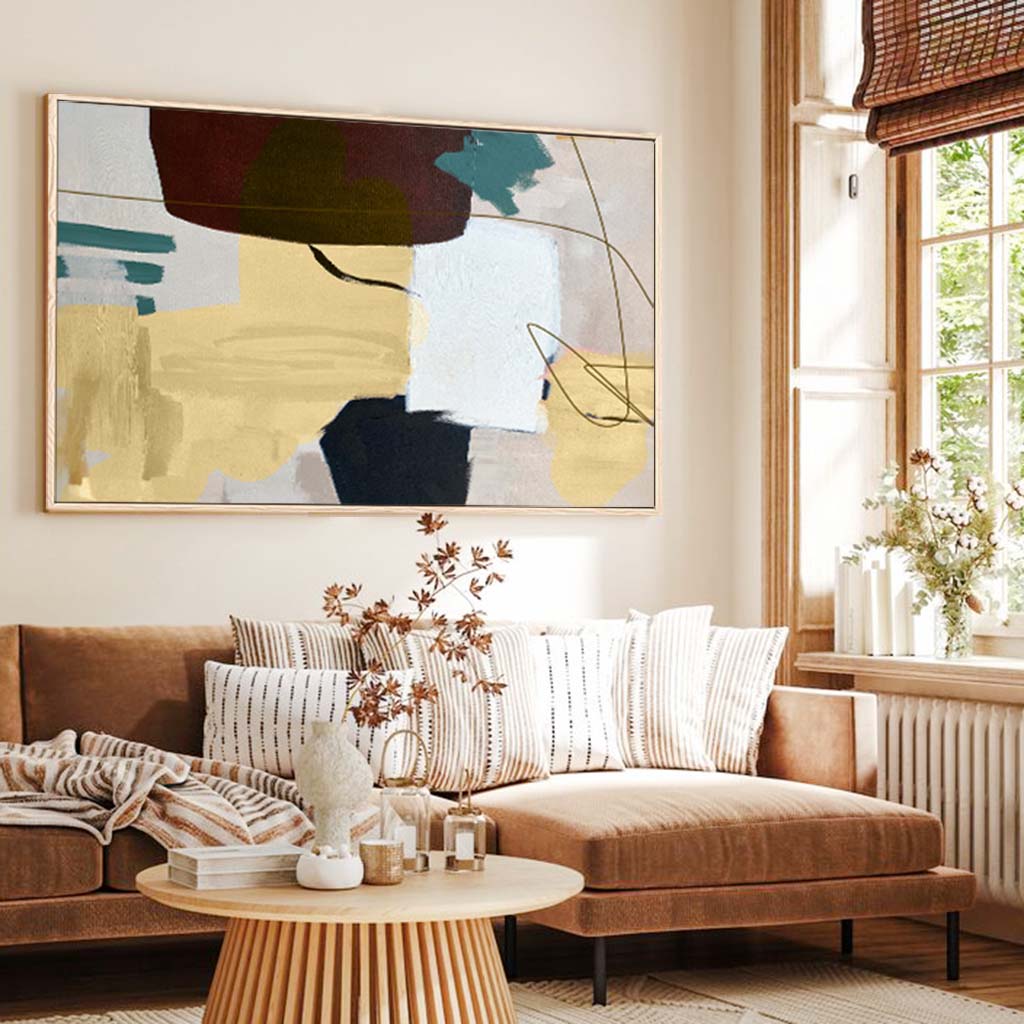This photograph captures the cozy and stylish ambiance of an indoor living room or den. The room features cream-colored walls that serve as a subtle backdrop for a large, rectangular piece of abstract artwork. This artwork, framed in beige, brings together hues of dark browns, creams, yellows, teal, black, and green, providing a striking focal point above a modern, retro-style sectional couch. The camel brown velvet sectional includes a chaise lounge and two clearly defined seats, adorned with decorative throw pillows in alternating vertical cream and white stripes, and a striped throw blanket in shades of brown and light beige. 

In front of the couch is a small, round coffee table with various muted brown accessories, including a dried floral arrangement, a small vase, perhaps a bottle of perfume, and a couple of books with white covers. The living room has hardwood floors mostly covered by a cream-colored rug, adding to the room's warm atmosphere. To the right, a bay window allows natural sunlight to stream in, giving the impression of late morning or early afternoon light. The window sill holds a bouquet of flowers and more white-covered books, while a white radiator below the sill contrasts with a wicker-style shade trimmed in wood. Through the window, one can see the hint of a tree outside, enhancing the room's serene vibe.